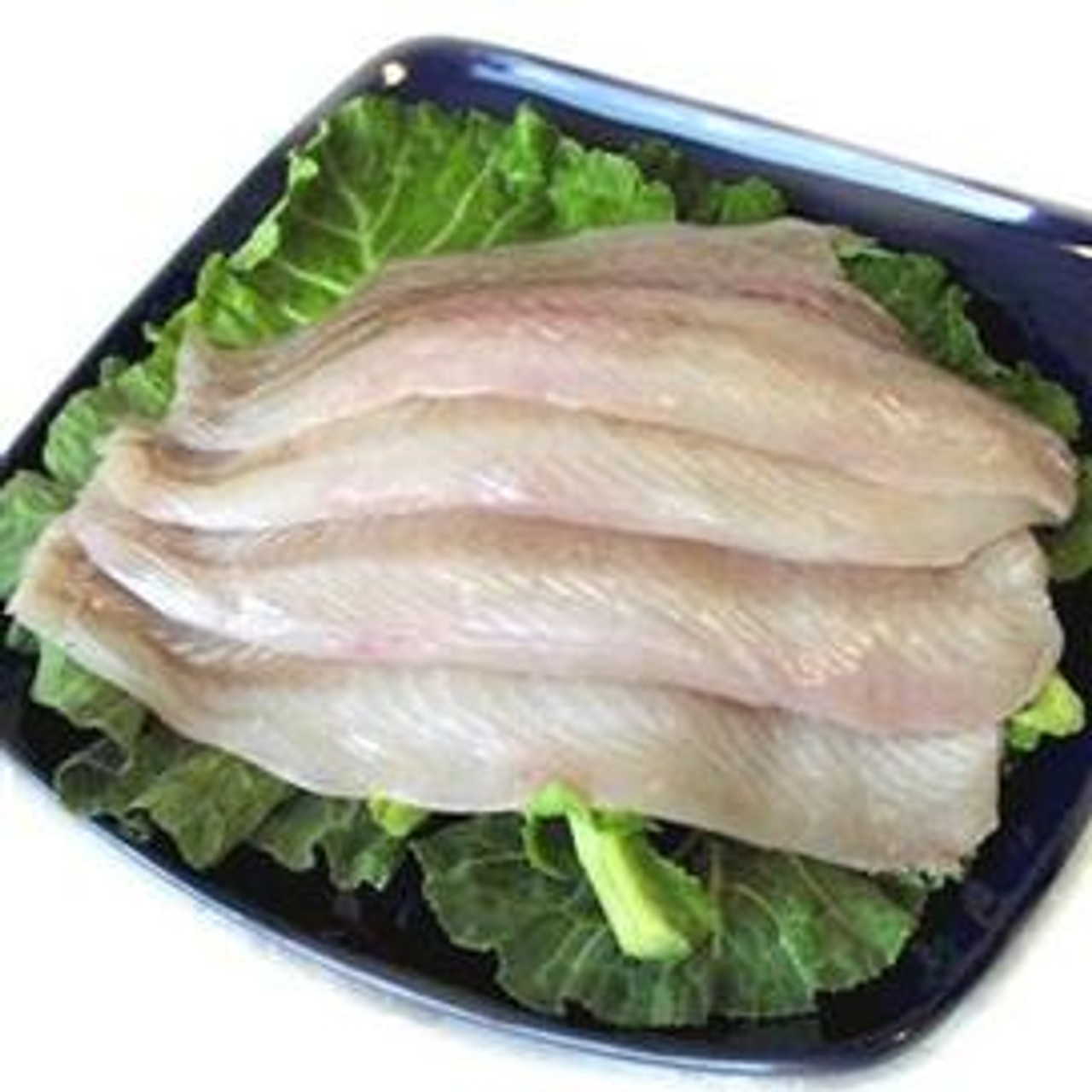This photograph showcases a shallow, metallic plate with light blue edges and a darker blue or black base, reflecting a hint of top light to reveal its true color. The plate has a rounded-square shape and is set against a stark white background, emphasizing the colors and textures within. The dish holds a dark green bed of leafy vegetables, which appear to be kale. Nestled on top of this bed are four long, slender fish fillets, arranged neatly. These fillets are uncooked, displaying a delicate white color with hues of pink and light tan, suggesting a type of white fish. The combination of the dark plate, green kale, and light-hued fish creates a visually striking composition.